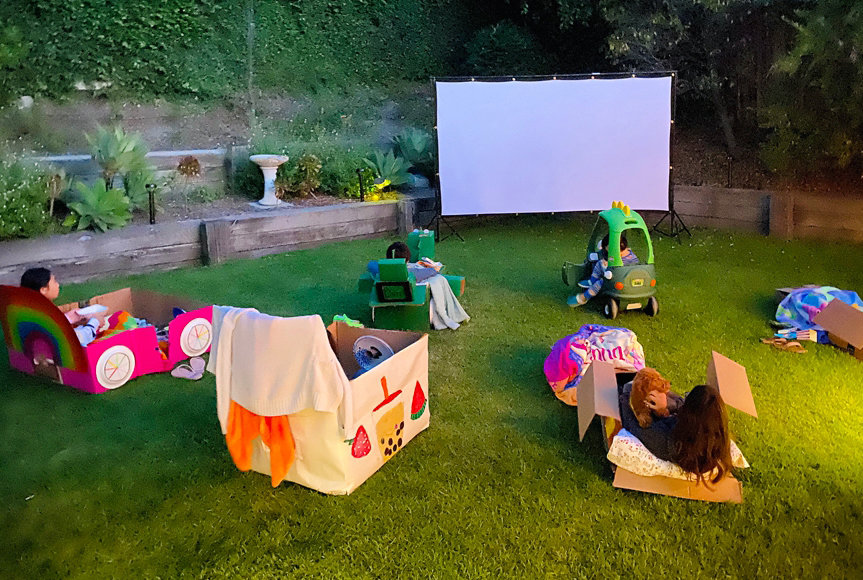This horizontally aligned rectangular picture captures a charming backyard movie night scene for children. The lower portion of the image features a lush green lawn, transitioning into a short retaining wall made of weathered wood, composed of three wooden planks stacked horizontally. This wall separates the grassy area from a garden bed filled with mulch, plants, and a birdbath statue. Above the retaining wall, various green bushes and trees frame the upper part of the scene, creating a cozy, enclosed atmosphere.

To the upper right of the image, a large white projector screen with a black outline and stand is on, suggesting the children are about to watch or are watching a movie. Scattered across the lawn are children seated in an assortment of creatively decorated cardboard boxes and toy vehicles, mimicking makeshift seats for their outdoor cinema.

In the lower left corner, a little girl with dark hair is seen from behind, holding a stuffed animal and sitting in a plain brown cardboard box. In the middle of the lawn, a large box draped in fabric and painted with vibrant fruits like strawberries and watermelons serves as the seat for another child. To the left, a brightly colored rainbow box, detailed with red, yellow, blue, and pink hues, holds another child. Additionally, there is a colorful bead cushion visible nearby.

On the far left side, another child sits within a rainbow-colored box, adorned with pink, white, orange, and green accents, sporting blue shoes. Further to the right, a child with dark hair and dressed in gray sits in a plain brown box, holding a brown stuffed animal. Another child to the far right is seated in a plain brown box with a blue and purple blanket.

In the foreground, two more children are visible. One is riding a green dinosaur toy, wearing a blue shirt, and draped with a white blanket. The other is in a toddler car with a green roof and a yellow spiky top, getting out of the vehicle, dressed in a blue and white outfit with matching slippers.

Overall, the scene is an idyllic snapshot of a backyard transformed into a whimsical movie night venue for kids, surrounded by greenery and playful, homemade seating arrangements.